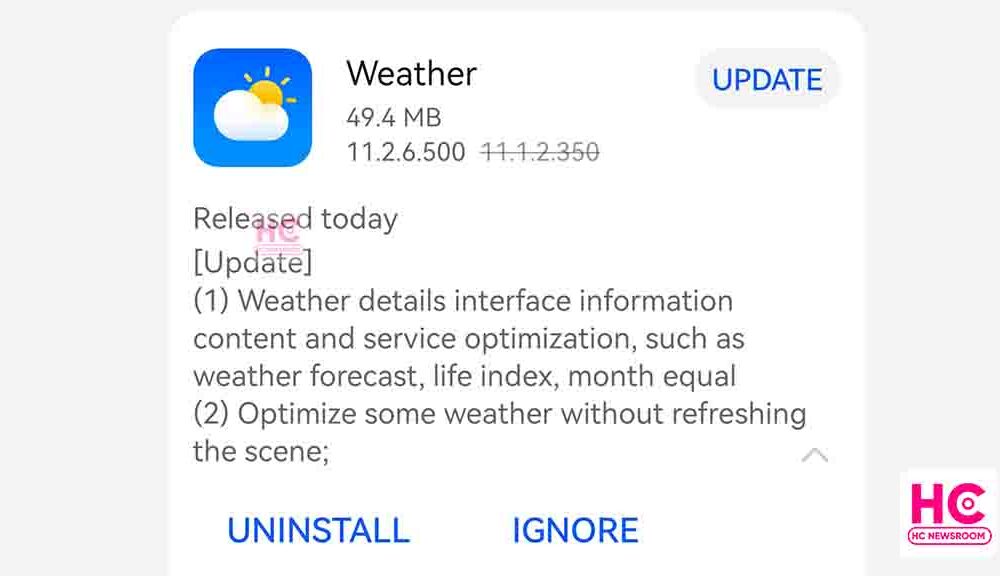The image depicts a weather update page on a website. The interface is seen on a light gray background, likely indicating it is being viewed on a desktop rather than a mobile phone as there are no icons at the top. 

At the top of the page, in large black letters, it reads "Weather," accompanied by a small blue square that features a partially cloudy icon with a sun. To the upper right corner, there is a notification for an update, with "UPDATE" written in blue uppercase letters, enclosed within a gray box.

The update information displayed includes the size, "49.4 MB," and the current version "11.2.6.500," with the previous version "11.1.2.350" crossed out. Additionally, it mentions that this release was made available today, with a faint watermark from "HC Newsroom" indicating its source. Bracketed text also includes the word "update."

The detailed update highlights include: 
1. Enhancements in the weather details interface.
2. Improvements in information content and optimization of services, such as the weather forecast and life index features, ensuring dynamic updates without requiring a page refresh.

Below these details, there are two prominent buttons, both in large blue capital letters: "UNINSTALL" and "IGNORE."

Along the right side of the page, there is a hot pink text that reads "HC Newsroom," indicating the origin of the weather update information.